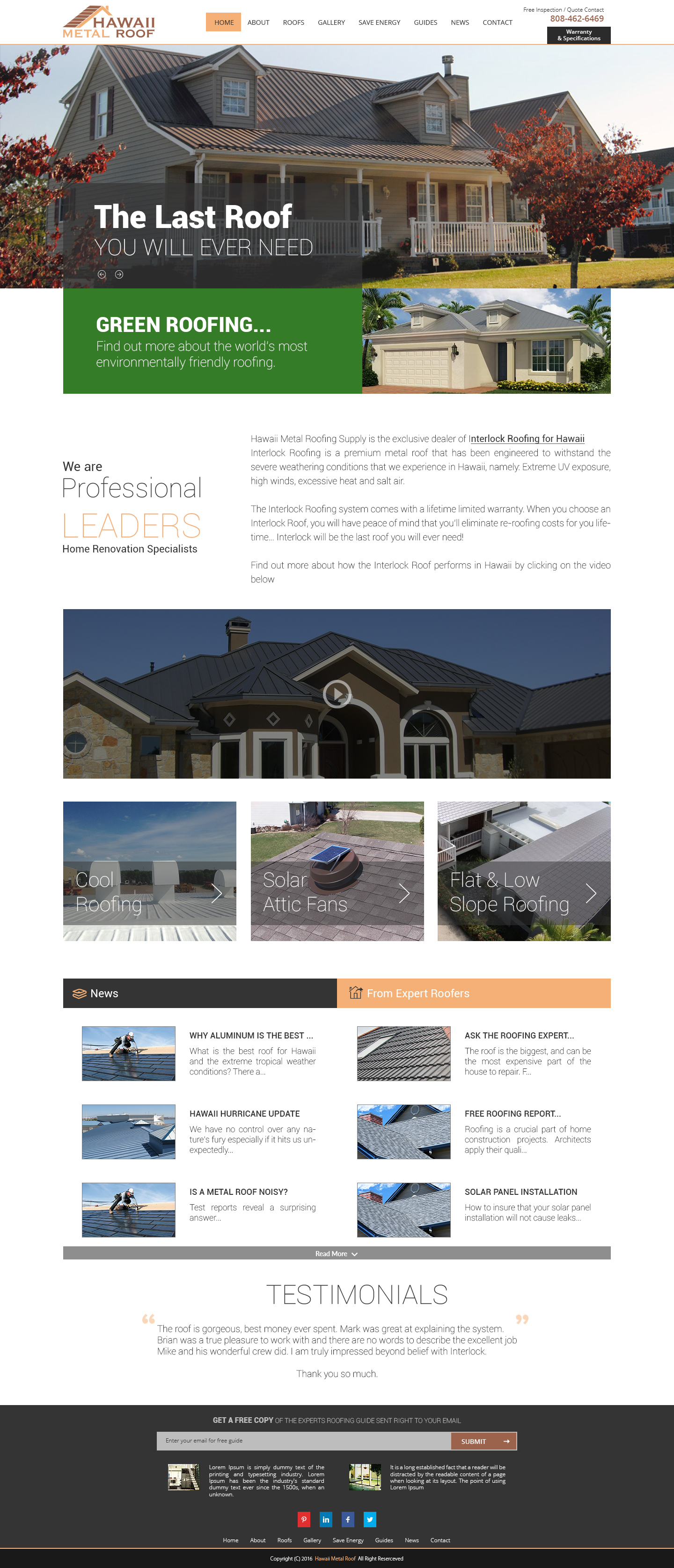The image depicts a comprehensive screenshot of a website dedicated to green roofing solutions. It showcases a full-length webpage starting from the top, highlighting a pristine white metal roof on a two-story single-family home. The top left corner of the image features this immaculate roof set against a clear sky, underscoring the website’s core subject.

At the very top of the screenshot is a navigation menu containing eight buttons neatly arranged for easy access. The buttons are labeled as follows: Home, Layout, Picture, and other additional options, which cater to the various sections of the site. 

Dominating the top section of the website is a banner displaying an image of the aforementioned single-family home. The house, sporting its white metal roof, exudes an air of modernity and sustainability. Towards the bottom left corner of this banner image, a bold text overlay proclaims, "This is the last roof you will ever need." This statement is rendered in striking white text, complemented by a subtle gray overlay beneath it to enhance readability.

Directly below this assertive tagline is a smaller, vibrant green rectangle containing the words "Green Roofing," emphasizing the eco-friendly aspect of the roofing solutions offered. This detailed layout effectively captures the key elements and navigation structure of the website, guiding users through its features with clarity and visual appeal.